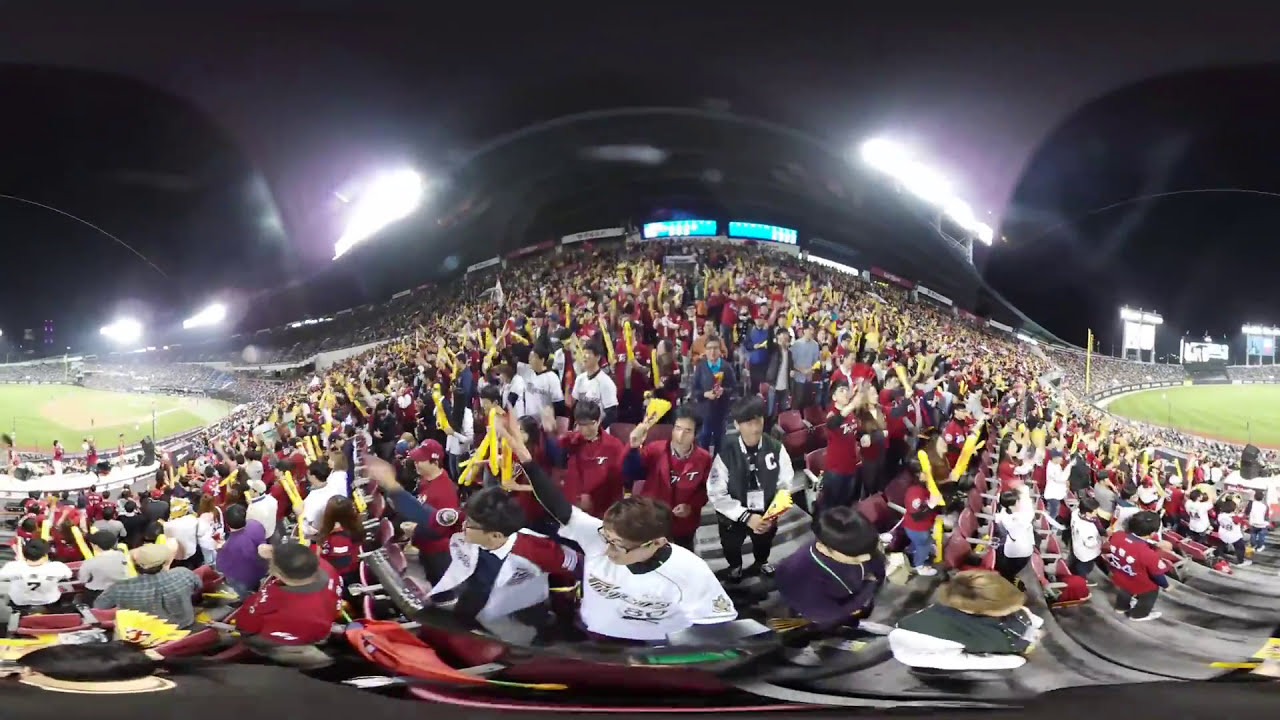The photograph captures a nighttime sporting event, most likely a baseball game, viewed through a fisheye or wide-angle lens that creates a distorted, cylindrical effect. The image showcases a stadium packed with an enthusiastic crowd, predominantly dressed in red and waving yellow flags. The seating area, enveloped in a bell-curve shape, stretches from the lower left to the lower right corner, arching upward in the center where it is filled with cheering fans. The field appears divided: the left side features a visible baseball diamond, while the right side is characterized by outfield green and prominent billboards. A dark sky, punctuated by field lights, forms the backdrop of this vivid scene, accentuating the energy and dynamism of the event and its supporters.